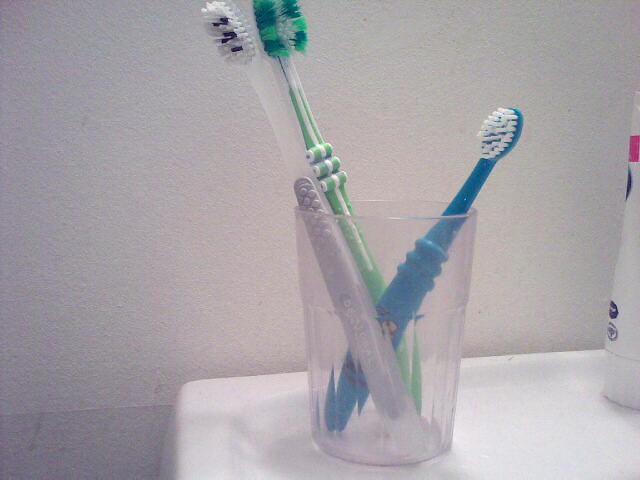This is a color photograph taken in a bathroom, showcasing a clear, slightly opaque plastic glass on a white, tray-like bathroom vanity. Inside the glass, three toothbrushes are visible: one with a grey handle and a clear head featuring white and black bristles; a second toothbrush with a green and white striped handle and green, blue, and yellowish-green bristles; and a smaller, kid's toothbrush with a blue handle and white bristles. To the right of the glass, a bottle with a red cap and partially visible blue or black writing can be seen, identified possibly as a tube of toothpaste. The background is a grey wall, with indistinct grey lines suggesting possible tiling at the bottom.